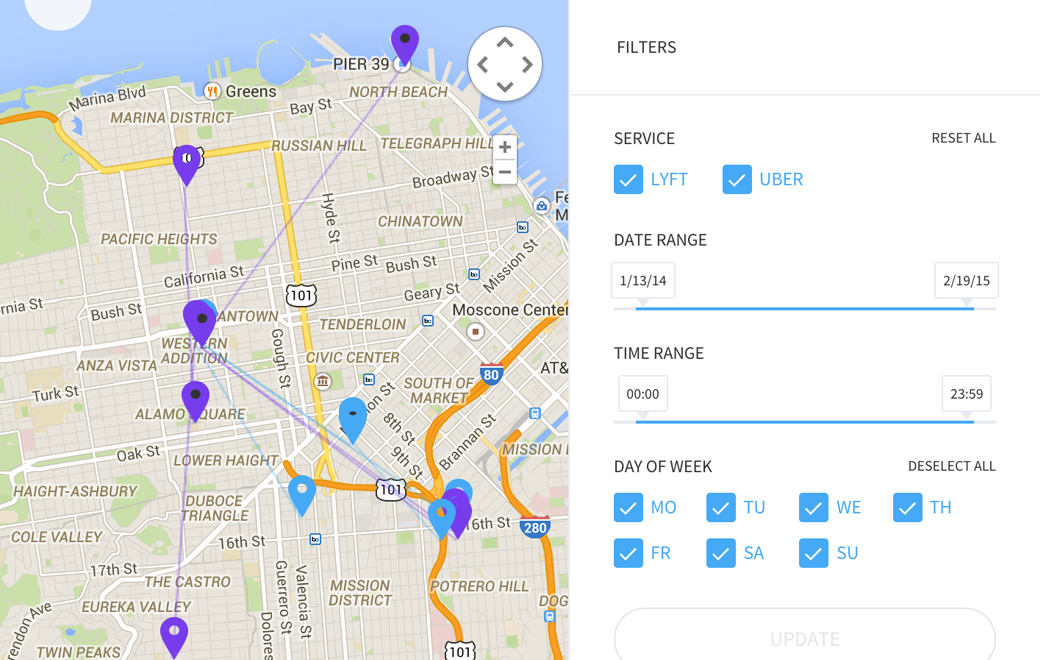A detailed map displays a waterfront area with several prominent landmarks and highways. Purple and blue pins are scattered across the map, though their purposes are unclear. The map features numerous Spanish-named locations, Marina Boulevard, and Pier 39 prominently at the top. I-80 and I-280 appear, providing major road connections, and US Highway 101 is also visible intersecting the region. A notable Chinatown area is marked, suggesting the city could be San Francisco, given the layout and prominent features.

The map also includes filters indicating a search for rideshare services, specifically Lyft and Uber, with a date range from January 13th to February 19th, 2015. The search parameters cover a 24-hour period across all days of the week, possibly to estimate ride availability and distances within this timeframe. The purpose of the purple and blue pins remains uncertain, as they do not clearly correspond to the two rideshare services.